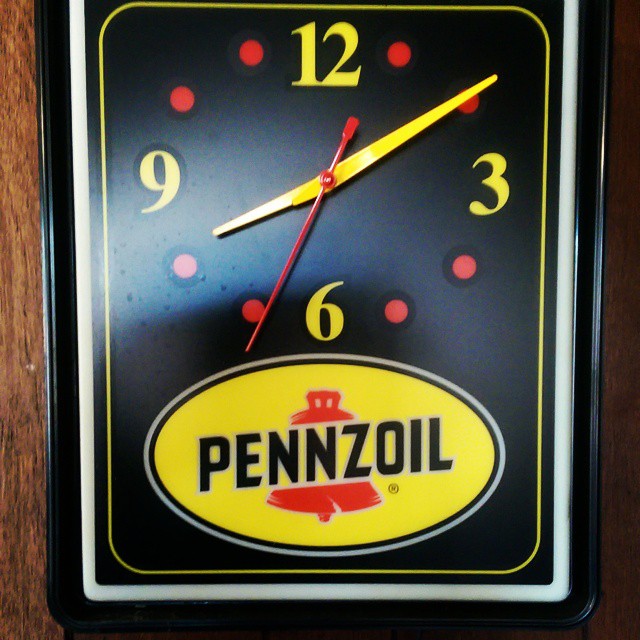This image depicts a distinctive rectangular black clock hanging on a wall adorned with wood paneling. The clock features a black face accented by yellow minute and hour hands, and a contrasting red second hand. The time is displayed using yellow numbers at the 12, 3, 6, and 9 o'clock positions, with two red dots marking the intervals between each of these numbers. At the bottom of the clock, there's a yellow oval with a white ring around its edge. The word "Pencil" is prominently inscribed in black within the oval, and it is flanked by small red bells positioned at the top and bottom. The clock is currently showing 8:10 and 34 seconds. Surrounding the entirety of the clock is a subtle white edging that frames its unique design.